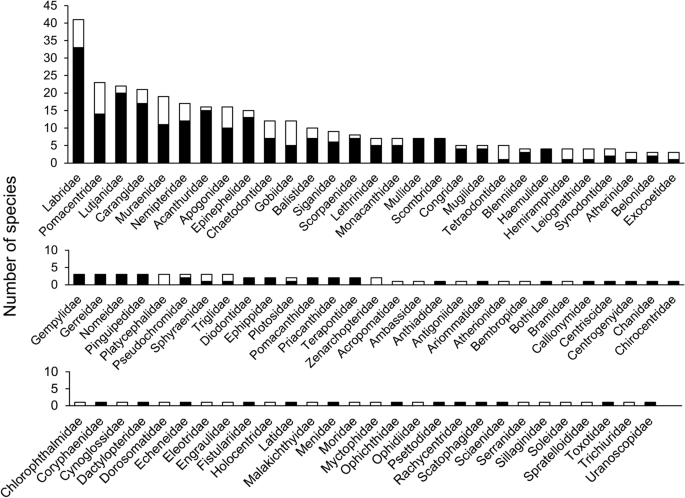The image consists of three vertically aligned bar graphs, each representing the number of species across various taxonomic families. The left-hand side of the image features a vertical axis labeled "Number of Species," ranging from 0 to 45 in increments of 5. The top bar graph shows a significant range of numbers, with the highest bar reaching nearly 40 species. The families represented here are Labiridae, Pumicentridae, Lutegenidae, Carangidae, Murinidae, Nemipteridae, Acanthuridae, Apogonidae, Epinephelidae, Chaetodontidae, Holocentridae, Balistidae, Siganidae, Scorpaenidae, Lethrinidae, Monacanthidae, Mullidae, Scombridae, Congridae, Muglidae, Tetraodontidae, Blenniidae, Haemulidae, Emmelichthyidae, Leiognathidae, Cynoglossidae, Atherinidae, Pleuronectidae, Pholidoteidae, and Exocoetidae.

The middle bar graph displays fewer species, with the largest bar only reaching around 5 species. Families included in this graph are Gempylidae, Gerreidae, Nomeidae, Plesiopidae, Apogonidae, Pseudochromidae, Serranidae, Triglidae, Diodontidae, Ephippidae, Pomacanthidae, Priacanthidae, Terapontidae, and Zanclidae. 

The bottom bar graph showcases very low numbers, with most species counts not exceeding 2. Families here include Cichlidae, Latidae, Echeneidae, Moridae, Menidae, Cyprinidae, Serranidae, Soleidae, Toxotidae, Trachinidae, Uranoscopidae, and several others. The entire image is in black and white, and the bars vary in height, emphasizing the variability in the number of species across different taxonomic groups.